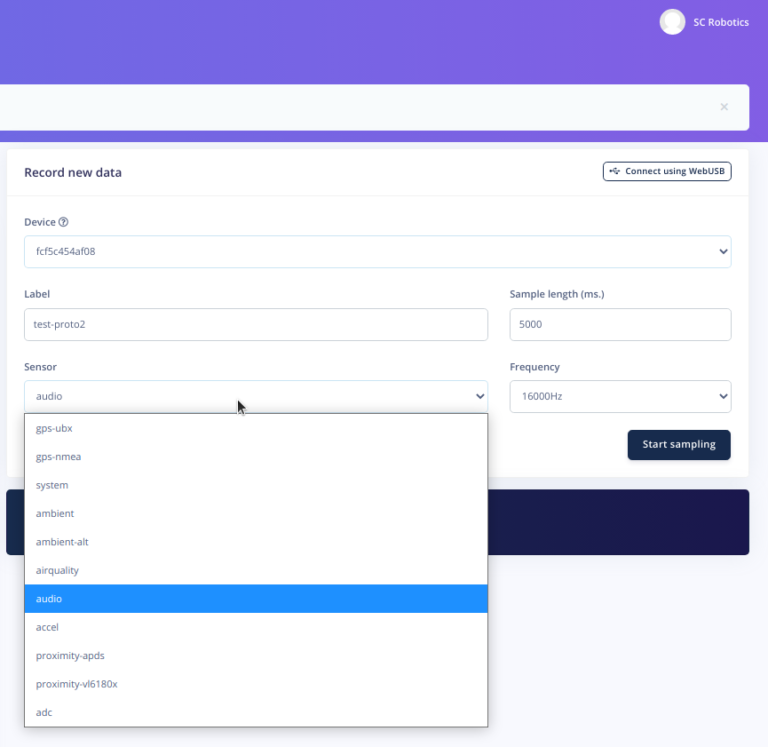The image displays an application interface from SC Robotics, characterized by a modern and user-friendly design. At the top right corner, the text "SC Robotics" is prominently displayed in white against a vibrant blue background. The main section of the interface features a clear, white backdrop that houses various input fields and options.

At the top of the body section, there is a prompt labeled "Record New Data," positioned to the left of a rectangular button that reads "Connect Using WebUSB." This button likely facilitates the connection of external devices via the WebUSB protocol.

Beneath this prompt, a series of labeled input fields are presented for the user to input specific data. The first field is titled "Device" and contains the pre-entered value "FCF5C454AF08." To the right of this field is a drop-down arrow, suggesting the availability of additional device options.

Following this, the next labeled field is "Label," which has the text "Test-Proto2" already entered, indicating a predefined label for the data set. Below this, the "Sensor" field is shown with the value "Audio" selected. This field also includes a drop-down menu, currently expanded to reveal other selectable sensor types, with "Audio" being the active choice.

Towards the bottom right corner of the interface, there is a prominent dark blue rectangular button labeled "Start Sampling," indicating the final action to initiate the data recording process. The overall layout is intuitive, with clearly defined areas for user input and actionable buttons, designed to streamline the data collection process for various applications in robotics.